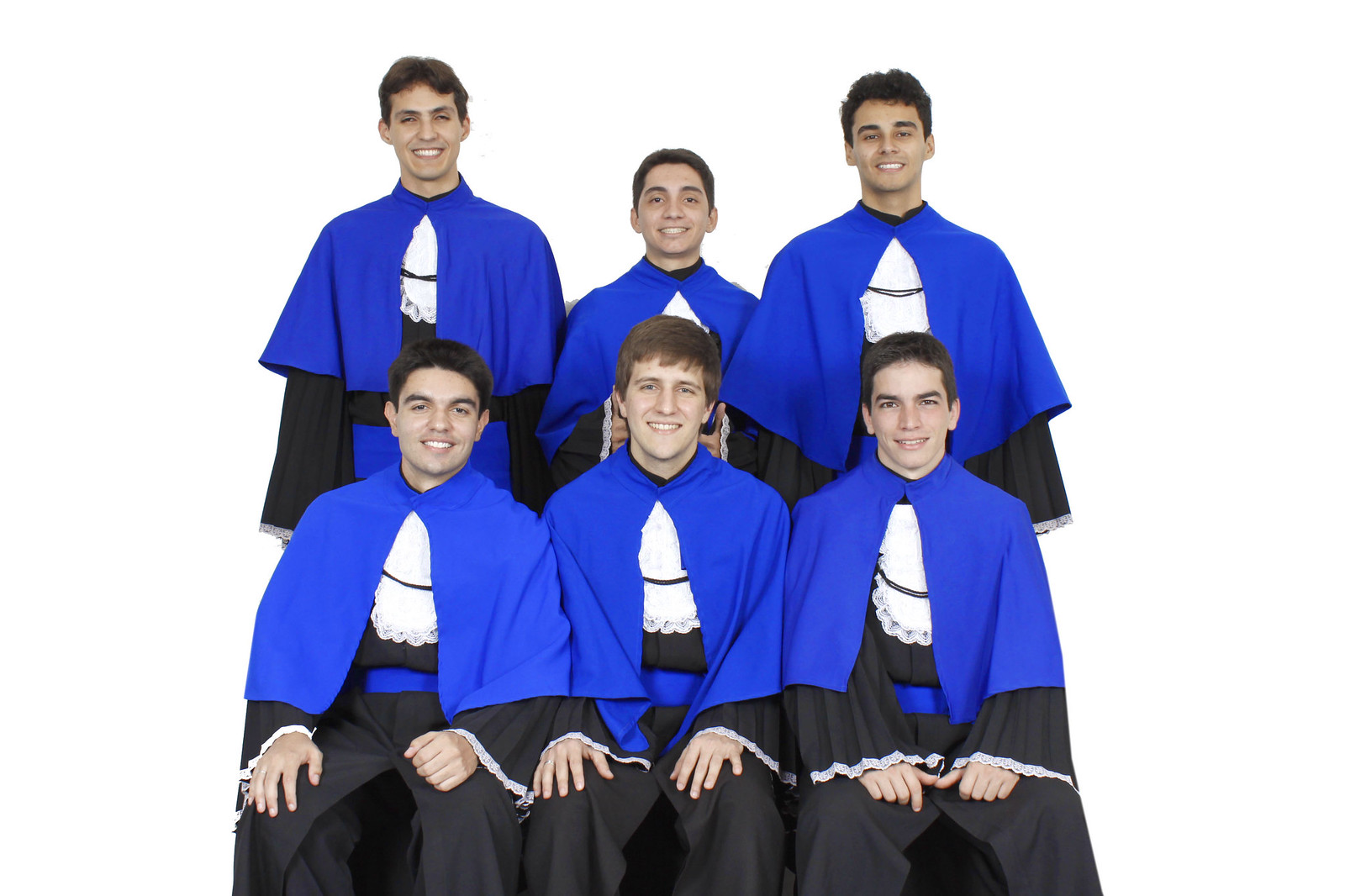This photograph captures a group of six young men, possibly a church choir or graduates, posed in two rows with three standing in the back and three sitting in the front. They all exude happiness with broad smiles on their faces. Each is dressed in a distinctive uniform comprising a blue cape with a large white collar, hemmed with white lace trimming, that overlays a black robe and black pants. The robes are cinched with a blue belt at the waist. Their hands are positioned uniformly—those in the front have their hands on their laps, while those in the back have their arms at their sides, except for the one in the middle, who holds an object partially obscured by another's head. The tallest individual is on the top left, while the second tallest is on the top right. The smallest stands in the center of the back row. The background is a simple white, bringing focus to the group's coordinated attire and cheerful expressions.